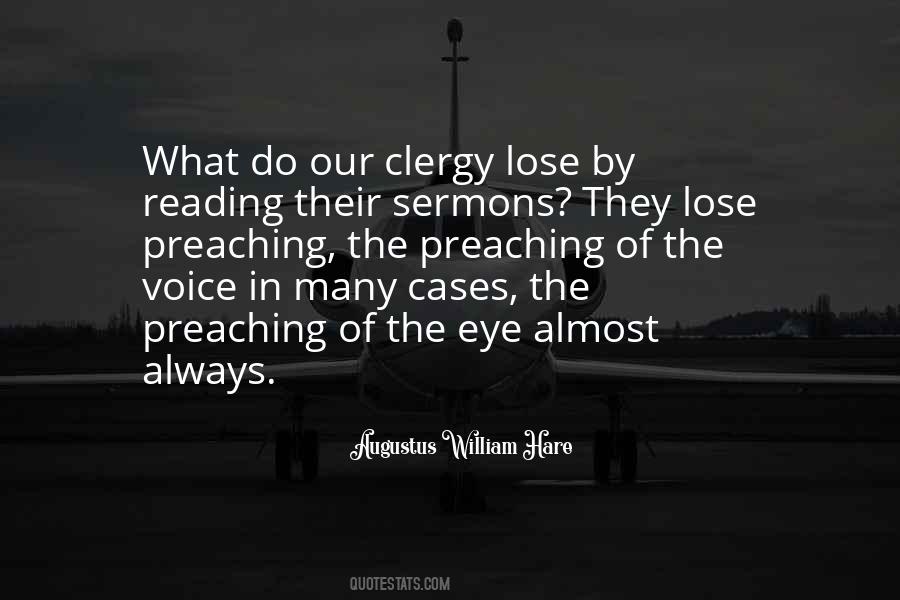The image features a white private jet facing directly towards the viewer, its nose closest to the camera and wings outstretched to either side, positioned on what appears to be an airport runway. The scene is largely void of color, presented in a grayscale palette with dark, muted tones, and some clouds visible in the sky. A tree line can be seen in the background.

Dominating the image is a text in white font that reads: "What do our clergy lose by reading their sermons? They lose preaching, the preaching of the voice in many cases, the preaching of the eye almost always." This quote is attributed to Augustus William Hare, with his name displayed below the text. Following his name are some indecipherable words written in a highly decorative, curly, and feminine font that might read "quotation" or possibly "quotes tats.com." Despite the challenging legibility, the text's prominent placement adds a reflective and thought-provoking element to the otherwise stark and somber image.